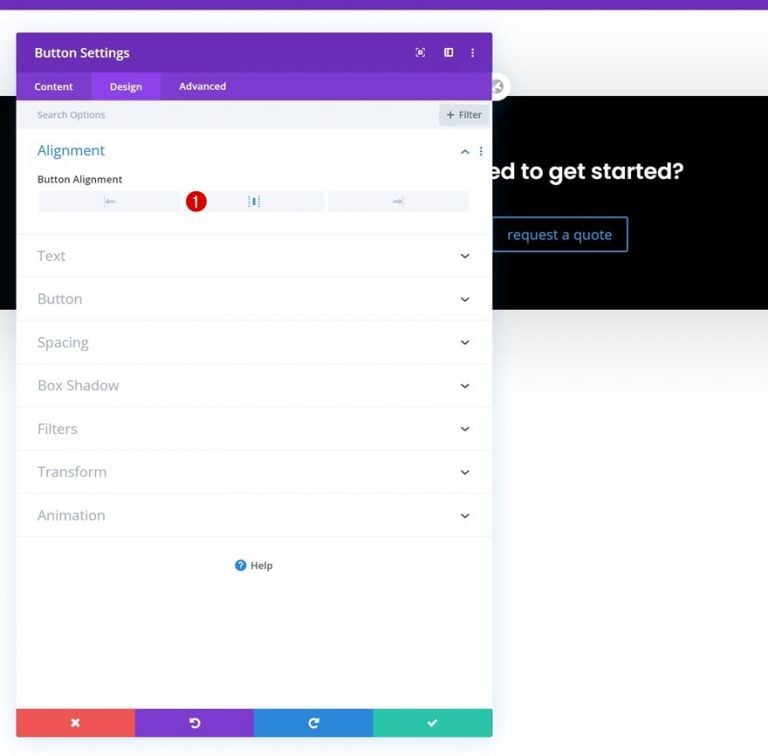The screen capture showcases a detailed user interface of a website or app, prominently featuring a pop-up window labeled "Button Settings." This pop-up is divided into three prominently displayed tabs: "Content," "Design," and "Advanced," though the interior of these tabs isn’t currently visible. Within these settings, options such as button alignment, resizing capabilities, and other design features like text, button spacing, box shadow, filters, transform, animation are listed, though not expanded.

Behind the pop-up, a partially obscured screen hints at additional instructional text ending with "...to get started?" and a "Request a Quote" button. The bottom section of the pop-up includes navigational and action buttons - a red "X" for closing, a green checkmark for confirming changes, and forward and back arrows for navigation. This comprehensive view indicates a robust set of customization tools for button design, albeit with some underlying instructions partially hidden by the pop-up.